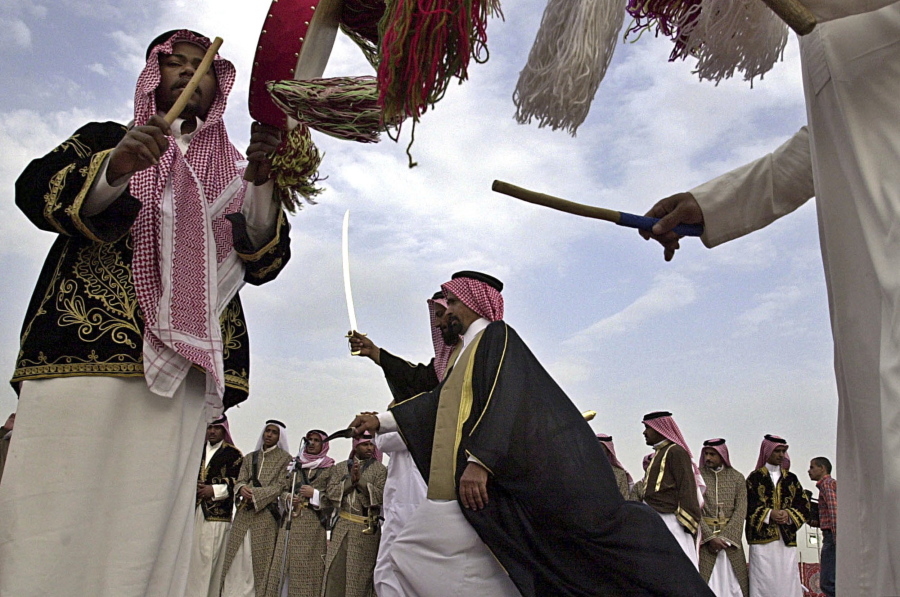This is a full-color, square photograph taken outdoors on a partly sunny day, depicting a lively celebration, possibly a parade or reenactment, involving Saudi Arabian men. The vantage point of the photo is from the ground pointing up at an angle, capturing a vibrant and dynamic scene.

In the center of the image, there is a man holding a sword aloft, wearing a long white cloak with a black cape over it, and an Arabian headpiece. Flanking him are two other men: one on the left sides appears to be wearing a white robe paired with a jacket, and he is playing a drum. Another man on the right, also in a white robe and traditional headgear, is holding a stick and possibly a tambourine. Encircling them is a line of onlookers, also dressed in traditional attire—ranging from white to olive-colored robes and some in what may appear as military garb. Some of these onlookers are holding various objects, including sticks and possibly drum-related items. The men’s headgear varies from pink and white to solid white, adding a colorful and cultural touch to the photograph. The atmosphere exudes a sense of rich cultural heritage and communal celebration.